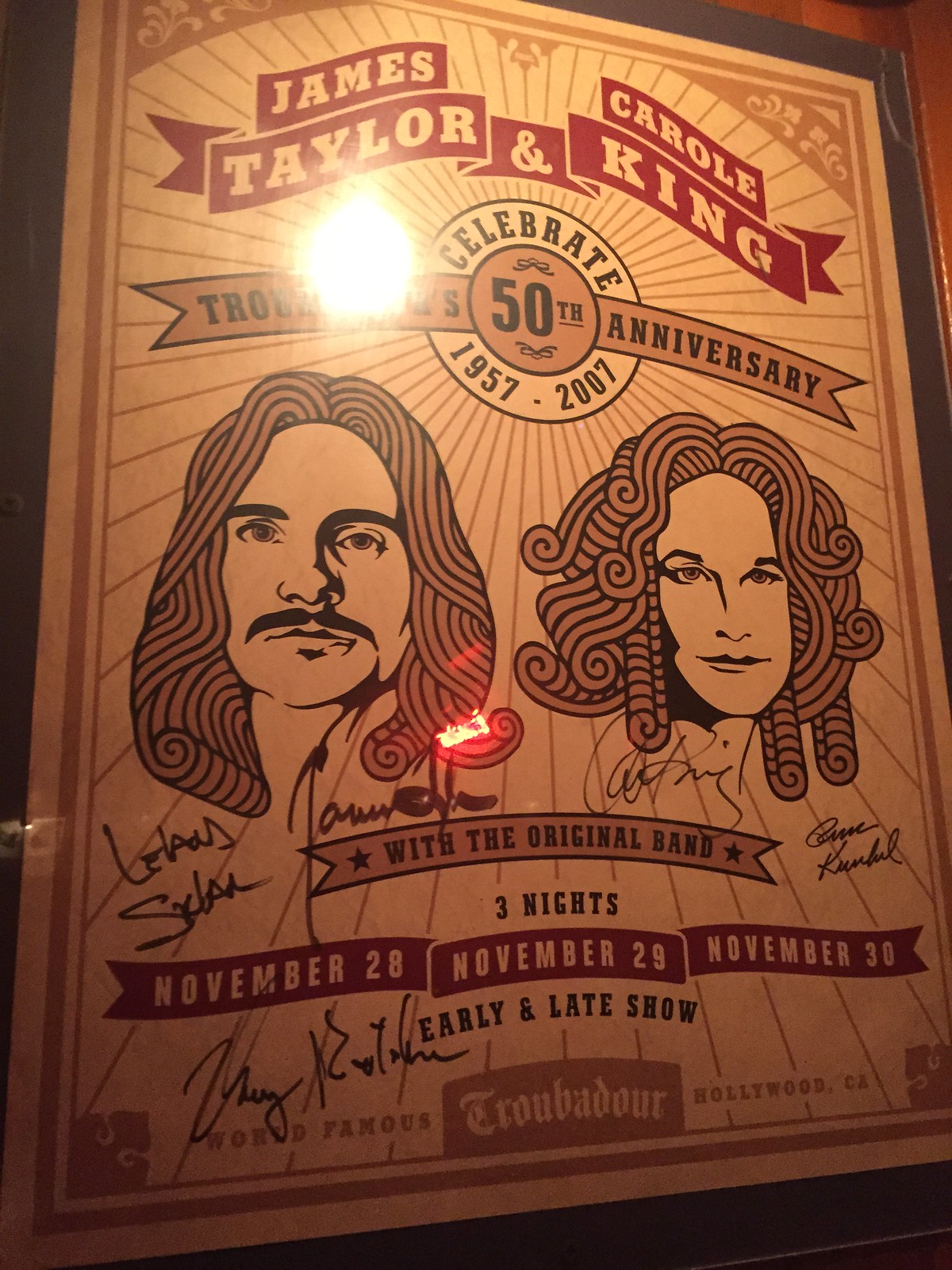The image is a detailed advertisement poster for a celebratory 50th anniversary concert featuring renowned musicians James Taylor and Carole King. The design is reminiscent of a vintage circus show with a color scheme dominated by shades of brown, off-white, beige, and red. The central figures, James Taylor and Carole King, are illustrated in a way that faces the viewer, capturing attention with their autographed signatures. The poster prominently lists three concert dates: November 20th, 28th, and 30th. The artistic style suggests a nostalgic, print-created look, emphasizing the long-standing legacy of the original band.